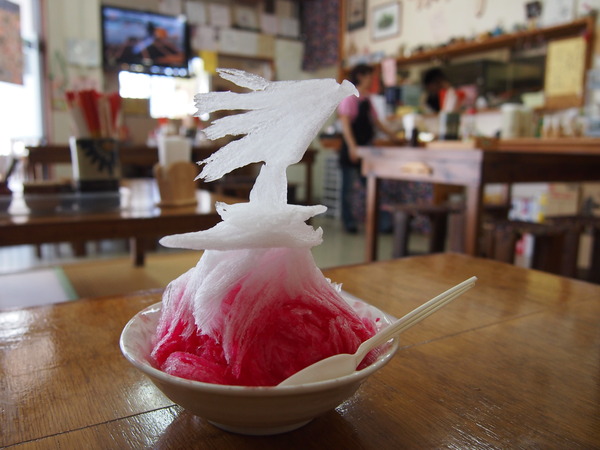In the image, a white bowl containing a red, gooey, ice-like dessert sits on a polished brown wooden table. Embedded in the bowl is a white plastic spoon resting against the red substance. Atop the red dessert is a striking ice sculpture resembling a bird standing on a platform, adding a decorative touch. The white bowl and its intricate contents are surrounded by more tables with various items strewn about. The background reveals a bustling scene with people, a concession stand area, a TV screen on the far wall, and various pictures adorning the walls, enhancing the lively ambiance.